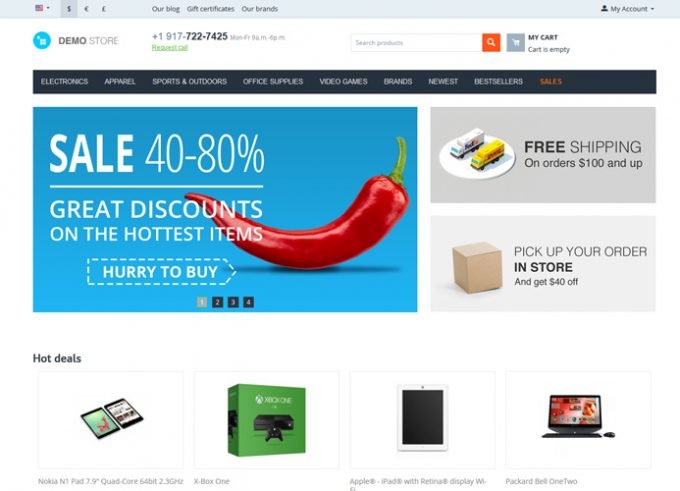The screen capture depicts a detailed e-commerce webpage layout. At the top, a thin gray navigation bar features several icons: an American flag, a dollar sign, a bell, and one more too blurry to identify. Alongside these are links labeled "Our Blog," "Gift Certificates," and "Our Brands." On the right side of the bar, there is a black silhouette icon with a head and shoulders marked "My Account" with a drop-down arrow. Adjacent to this are a blue and white circle indicating "Demo Store" and a phone number, 1-917-722-7425, followed by a gray, blurry text.

Below, green text appears with a white and gray search box, housing an orange and white magnifying glass icon. The search bar is accompanied by a white and gray cart indicating "My Cart" with the text "Cart is empty."

A navy blue strip follows, containing white and orange text links to categories: Electronics, Apparel, Sports & Outdoors, Office Supplies, Video Games, Brands, Newest, Best Sellers, and a prominent orange "Sales" section.

The subsequent blue background displays a white text message next to a red chili pepper icon: "Sale 40-80% great discounts on the hottest items. Hurry to buy." Below this are numbered boxes from 1 to 4.

Further down, another section highlights "Free Shipping on orders $100 and up," featuring a white and yellow truck icon within a white circle. This is succeeded by a promotion: "Pick up your order in store and get $40 off," next to a cardboard box icon.

The "Hot Deals" segment showcases images of two black tablets labeled Nokia with specs "7.9 inch quad-core 64-bit 2.3 GHz," an Xbox One game console in black with green and white packaging, a white Apple iPad with a black screen, and an unspecified black computer.

Overall, the layout displays a mix of promotional graphics and product highlights, providing a comprehensive snapshot of the webpage offerings.